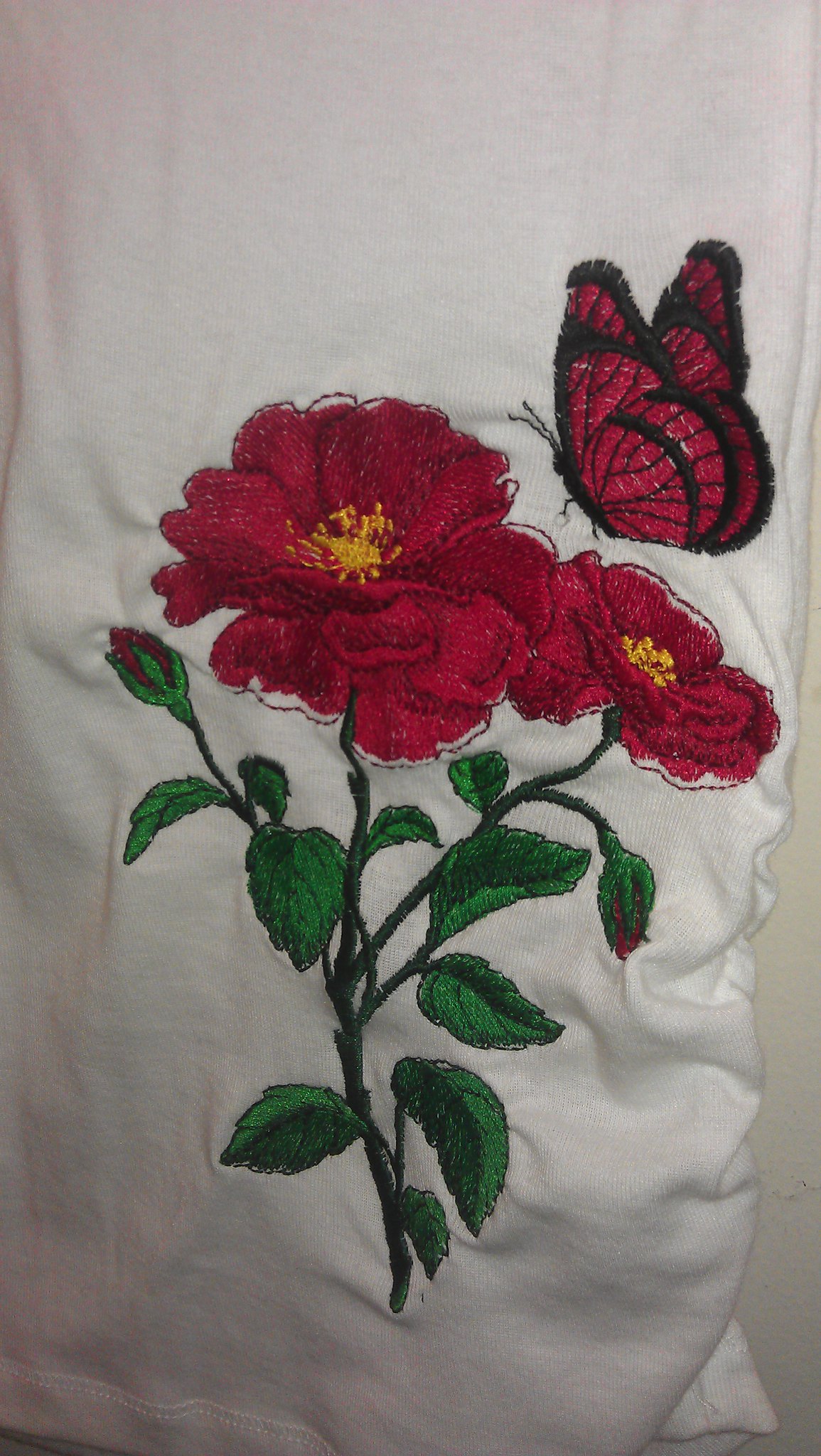The image is a rectangular photograph showcasing a white cotton fabric, possibly a pillowcase or a towel, with an elaborate embroidered design. The background is a solid bright white, and the embroidery features two prominent flowers attached to a single green stem. The flowers, one larger and one smaller, are deep red with a dozen or so petals and striking yellow centers. The green stem is adorned with emerald green leaves and a few unopened buds. To the top right of the image, a red butterfly with black-tipped wings and a black body appears to be hovering or about to land on the flowers, accentuating the detailed artistry of the embroidery. The butterfly's wings and body are finely detailed, with two black antennae and legs poised towards the flowers, adding a dynamic nature to the scene.